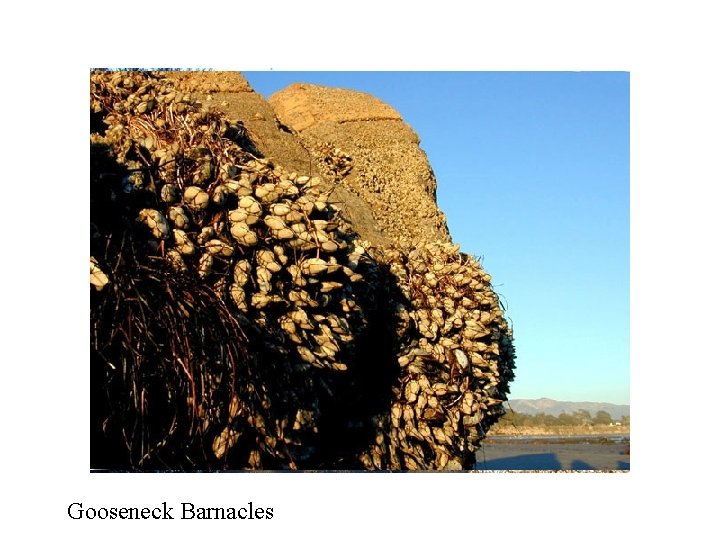The image depicts a cluster of Goose-neck barnacles hanging from a brown, rocky hillside, presumably exposed at low tide. These barnacles, beige in color and affixed to the stone surface, are identified by a label beneath the image reading "Goose-neck barnacles." In the background, you can see a sandy beach and receded waters under a bright blue sky. Intertwined with the barnacles are dark purple, root or stem-like structures, possibly a type of seaweed or sea plant, noticeable in the leftmost part of the picture.